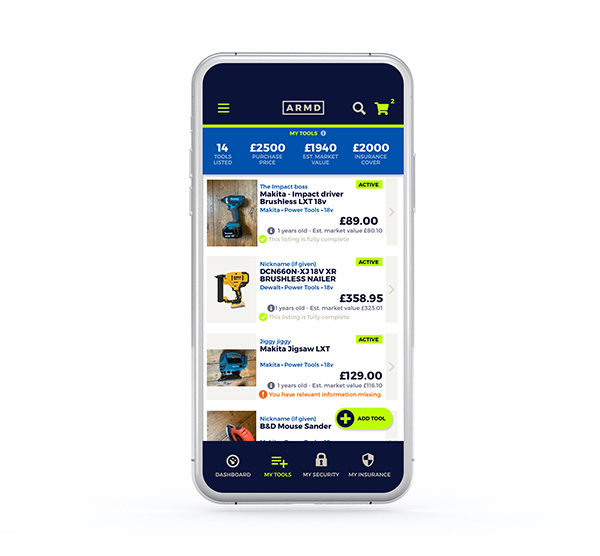A detailed screenshot of a smartphone app interface for managing tools and their insurance coverage. The screen displays four tool listings along with images and details, a navigation bar with four icons and labels at the bottom, and a top bar featuring the brand name, a search icon, and a cart icon. The header section lists key statistics: 14 tools, a purchase price total of £2,500, an estimated market value of £1,940, and insurance coverage of £2,000.

Below the header, the four listed tools are:
1. **Makita Impact Driver Brushless LXT 18-volt** priced at £89.
2. **DeWalt DCN660N-XJ 18-volt XR Brushless Nailer** priced at £358.95.
3. **Makita Jigsaw LXT** priced at £129.
4. **B&D Mouse Sander** with a prompt to add it.

Each tool listing has a status label on the right marked as "Active," and the tool images are positioned to the left of the text descriptions. At the bottom right corner of the last tool listing, there's a green plus sign icon for adding new tools.

The navigation bar at the bottom features icons labeled "Dashboard," "Tools," "Security," and "Insurance." The app interface has a modern, clean design with a white background that makes the text and icons stand out, creating a minimalist aesthetic.